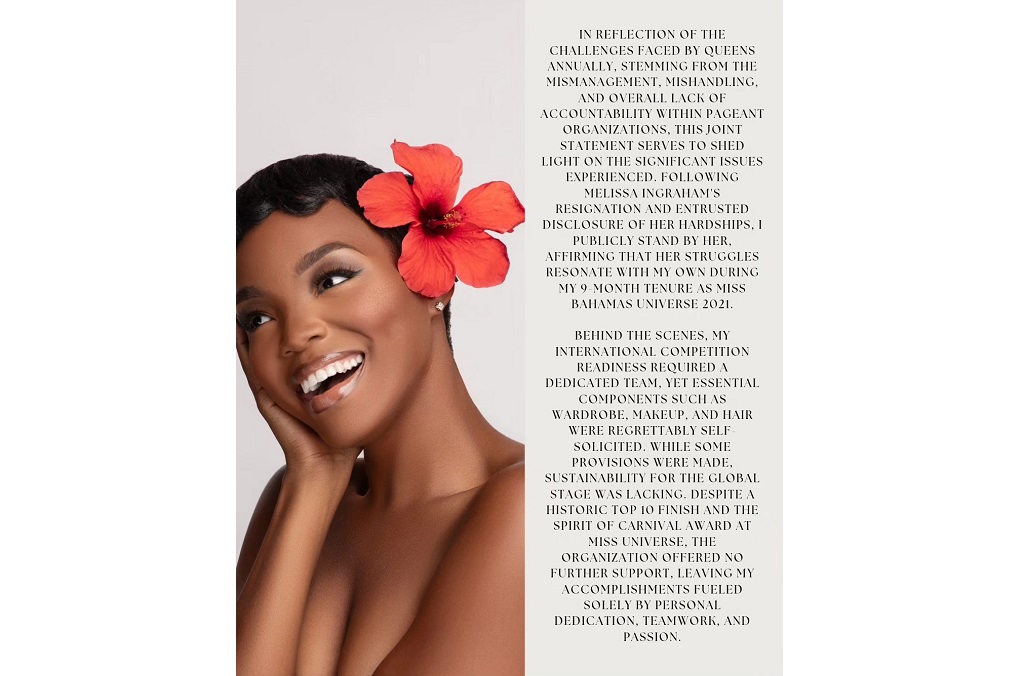The image features an African American woman with short, dark hair, adorned with a bright red lily tucked behind her ear. She is smiling warmly, resting her cheek and chin on her right hand, showcasing her perfectly shaped eyebrows and bright white teeth. The woman appears to be topless, though only her mid-forearm is visible, adding to the impression of bare shoulders. Her natural look is complemented by understated yet clearly applied makeup. 

To the right of her image, a column of text begins with, "In reflection of the challenges faced by Queens annually stemming from the mismanagement, mishandling, and overall lack of accountability within pageant organizations. This joint statement serves to shed light on the significant issues experienced following Melissa Ingram's resignation and her entrusted disclosure of hardships. I publicly stand by her, affirming that her struggles resonate with my own during my nine-month tenure as Miss Bahamas Universe 2021."

The text continues, detailing the unique challenges and lack of support encountered during her participation in international pageants, despite notable achievements such as a historic top ten finish and receiving the Spirit of Carnival award at Miss Universe. Essential components like wardrobe, makeup, and hair were self-solicited, as organizational support was insufficient for sustainable success on the global stage, leaving her accomplishments fueled solely by personal dedication, teamwork, and passion. The image and text together serve as a poignant advertisement or public service announcement highlighting these systemic issues within the pageant industry.